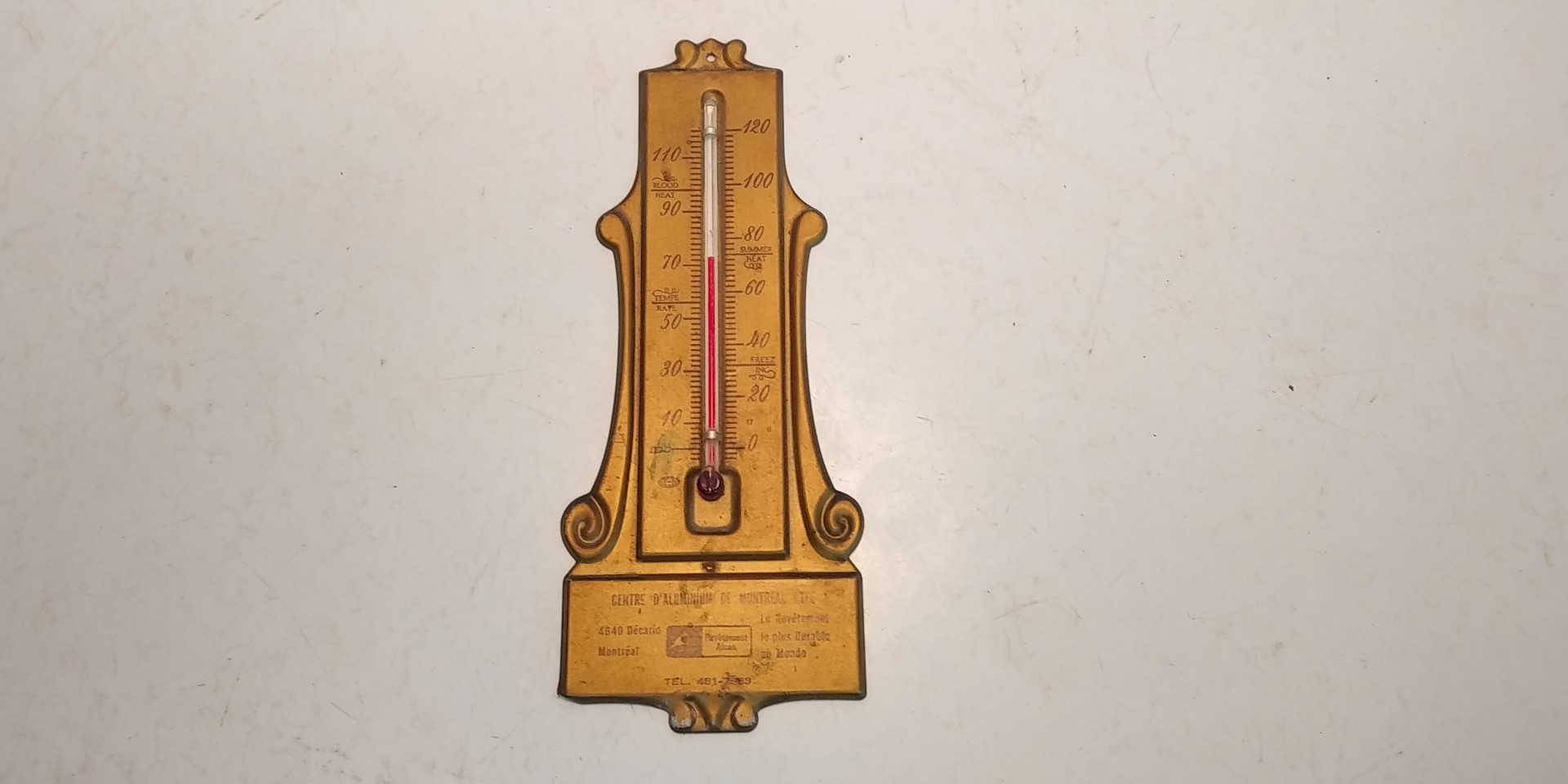The photograph showcases an intricately designed, vintage wooden thermometer mounted on an indoor wall, which is a subtle pale gray. The central focus, the thermometer, is well-lit, making it stand out against the lighter background. However, as your gaze moves towards the edges of the image, the wall fades into a darker shade of gray, creating a vignette effect that accentuates the central object.

The thermometer itself is crafted from wood with a warm, golden pine finish. It features ornate scrollwork designs that are either carved or wood-burned into its surface, adding a touch of rustic elegance. The wooden piece is primarily a vertical rectangle, and at its top, there is a small hole for hanging it securely on the wall.

At the heart of the design lies the thermometer, with a clear glass tube and a red mercury indicator showing the temperature at about midway up the scale. Below the scrollwork, there's a smaller, horizontal rectangle that likely contains the manufacturer's details or brand name, though the text is too small to discern clearly in the photograph.

The combination of the artistic woodwork, the functional thermometer, and the gentle gradation of the wall's color creates a visually appealing and nostalgic image that captures the essence of vintage craftsmanship.